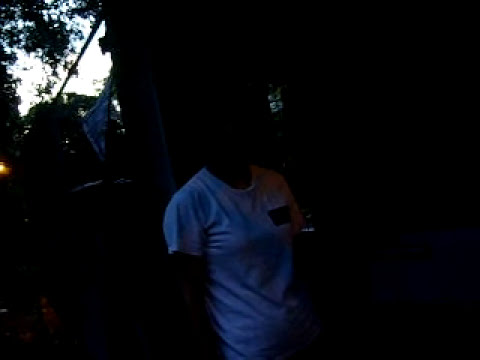In this predominantly dark and grainy outdoor image, the most discernible feature is a person wearing a white t-shirt standing in the center foreground. The individual, who appears to be female, is slightly turned to the right. The shirt has a bluish tint, likely due to surrounding light sources. Some dim daylight is visible in the top left corner, along with tree branches and what appears to be a yellow-white light source. Vaguely visible in the lower-left corner are some indeterminate light-colored objects, while a bit of sky and a possible cable and flag can also be faintly seen in the background. Overall, the image lacks clarity and detail, making it difficult to distinguish more specific features.